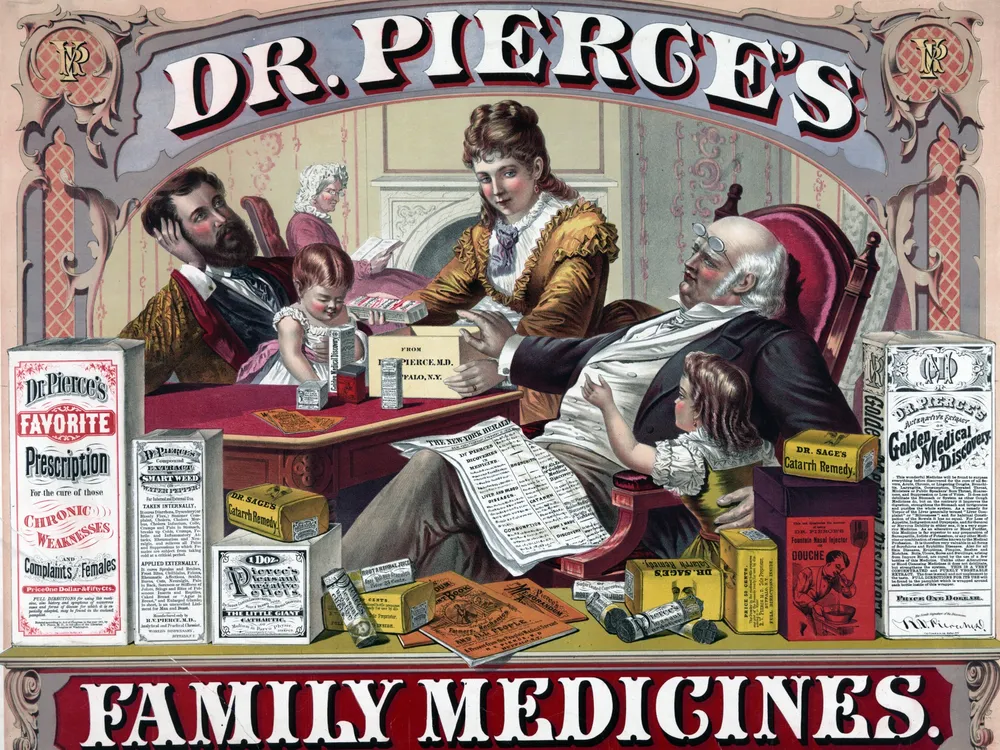This vintage-style advertisement, resembling a detailed painting from the late 1800s to early 1900s, promotes Dr. Pierce's Family Medicines. At the top of the image, a white text banner proudly displays "Dr. Pierce's," while the bottom features a red banner with "Family Medicines." The central illustration portrays a family seated around a green shelf laden with colorful, old-fashioned prescription boxes.

In the scene, a distinguished, mostly bald gentleman with white hair and large eyebrows sits on the left, dressed in a suit, and holding a child. A woman in a gold dress with a white top is engaged in unpacking a box, while another child stands nearby. Beside her, an elderly man, possibly the grandfather, sits with a newspaper and his arm around the child. In the background, an older woman with white hair, probably the grandmother, sits reading a book.

The family appears to be examining Dr. Pierce's various medicinal products, which include "Dr. Pierce's Favorite Prescription," primarily for chronic female complaints, "Smartweed Extract from Water Pepper," "Dr. Sage's Catarrh Remedy," and "Dr. Pierce's Pleasant Purgative Pellets." The entire advertisement exudes a nostalgic, Victorian-era charm, capturing a moment of intimate family interaction amidst the myriad of Dr. Pierce's marketed cures.